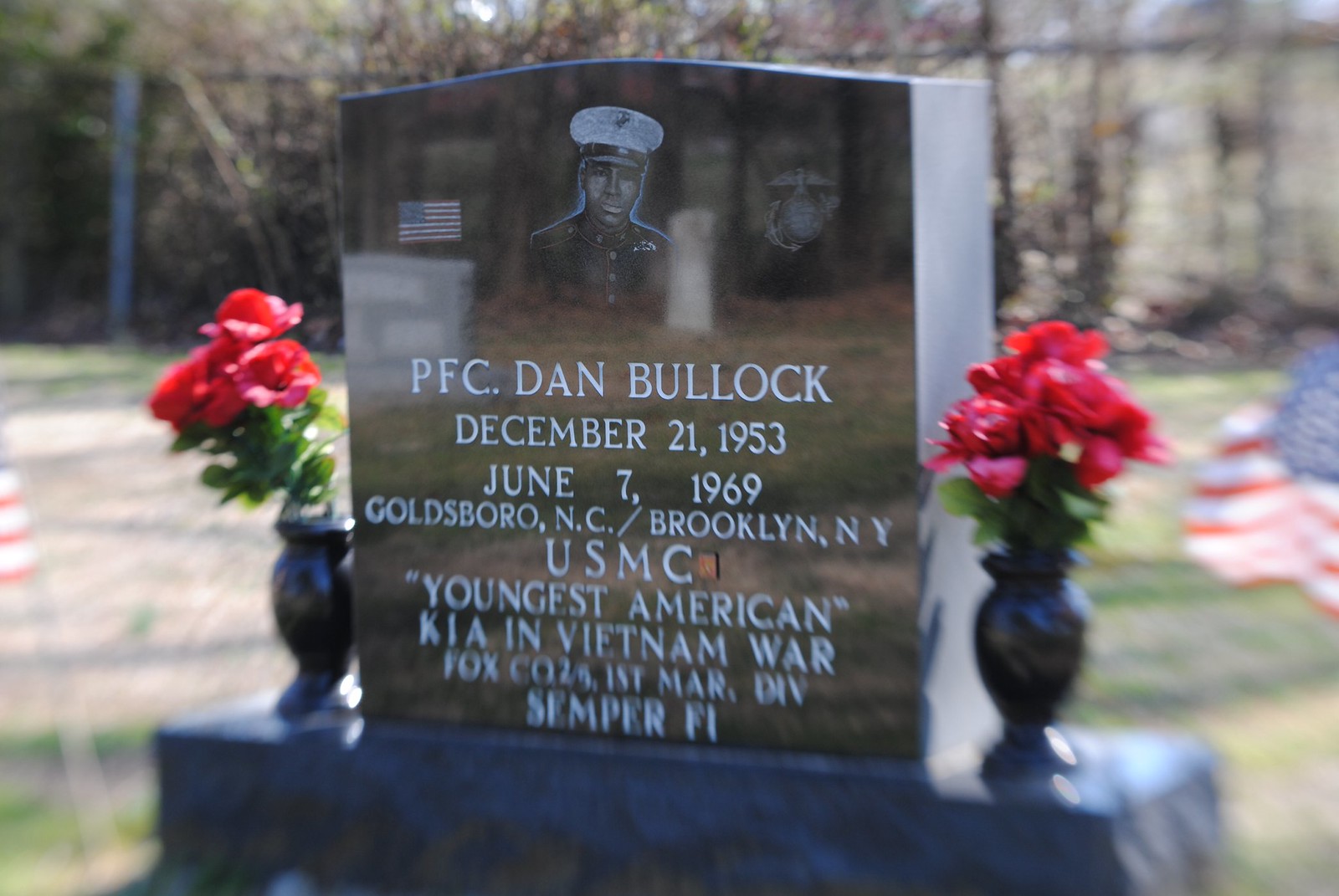This photograph captures the gravestone of Private First Class Dan Bullock, a soldier in the United States Marine Corps and the youngest American killed in action during the Vietnam War. The image, though blurry around the edges, prominently features a shiny, polished marble headstone with a rounded top. Engraved at the top of the gravestone is a photograph of PFC Dan Bullock in his Marine Corps uniform, complete with a white Marine hat and the USMC emblem on the right side. The text on the stone reads: "PFC Dan Bullock, December 21st, 1953 - June 7th, 1969. Goldsboro, North Carolina / Brooklyn, New York. USMC. Youngest American KIA in Vietnam War. Fox CO2, 1st March Division. Semper Fi." On either side of the gravestone are black marble vases filled with red tulips, and American flags are placed nearby, flanking the monument. In the background, a blurred fence and leafless trees can be seen, adding a somber atmosphere to the scene. Two bouquets of red roses also rest beside the grave, enhancing the solemnity and honor of the memorial.